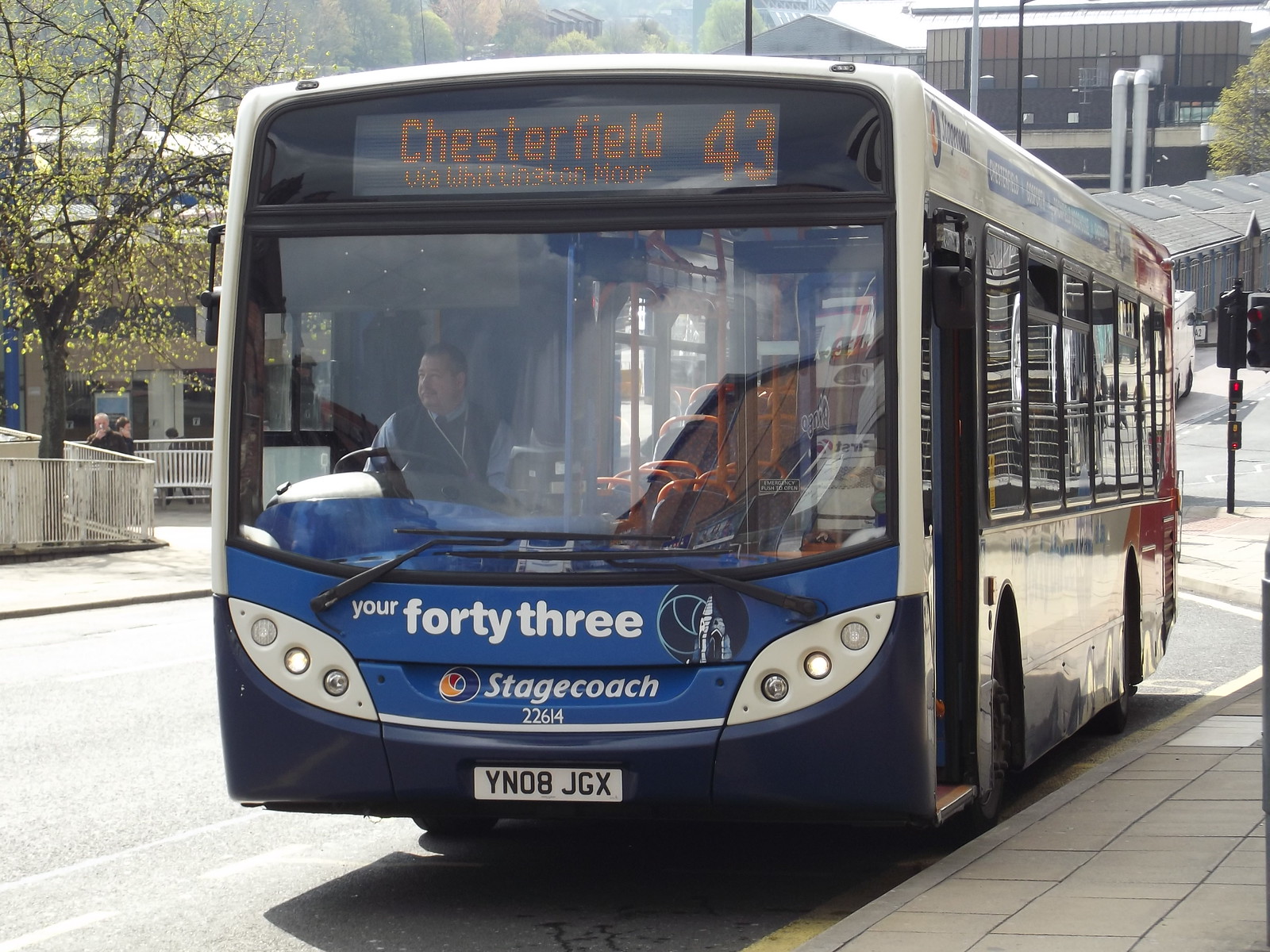In this detailed outdoor photograph taken in the middle of the day, a large passenger bus is prominently featured, parked at a curb on the side of an asphalt road. The bus, reading "Your 43, Stagecoach, 22614," with a license plate "YN08JGX," is clearly seen in the center of the image with no passengers inside, except for the bus driver seated at the wheel. Above the windshield, an electronic banner displays "Chesterfield 43 via Whittington Moor" on a yellow-on-black background.

To the right of the bus, another bus can be spotted in the background along with streetlights and various buildings and houses behind them. On the left side of the road, across from the bus, an area with benches, trees, and a few gathered people is noticeable. There's also a white fence surrounding a blooming tree in the upper left. The asphalt road is bordered by what appears to be a stone sidewalk in the bottom right corner. The scene is brought together with an array of colors including gray, white, yellow, tan, blue, orange, red, and green. The surroundings, comprising more buildings and some trees, suggest an urban environment.